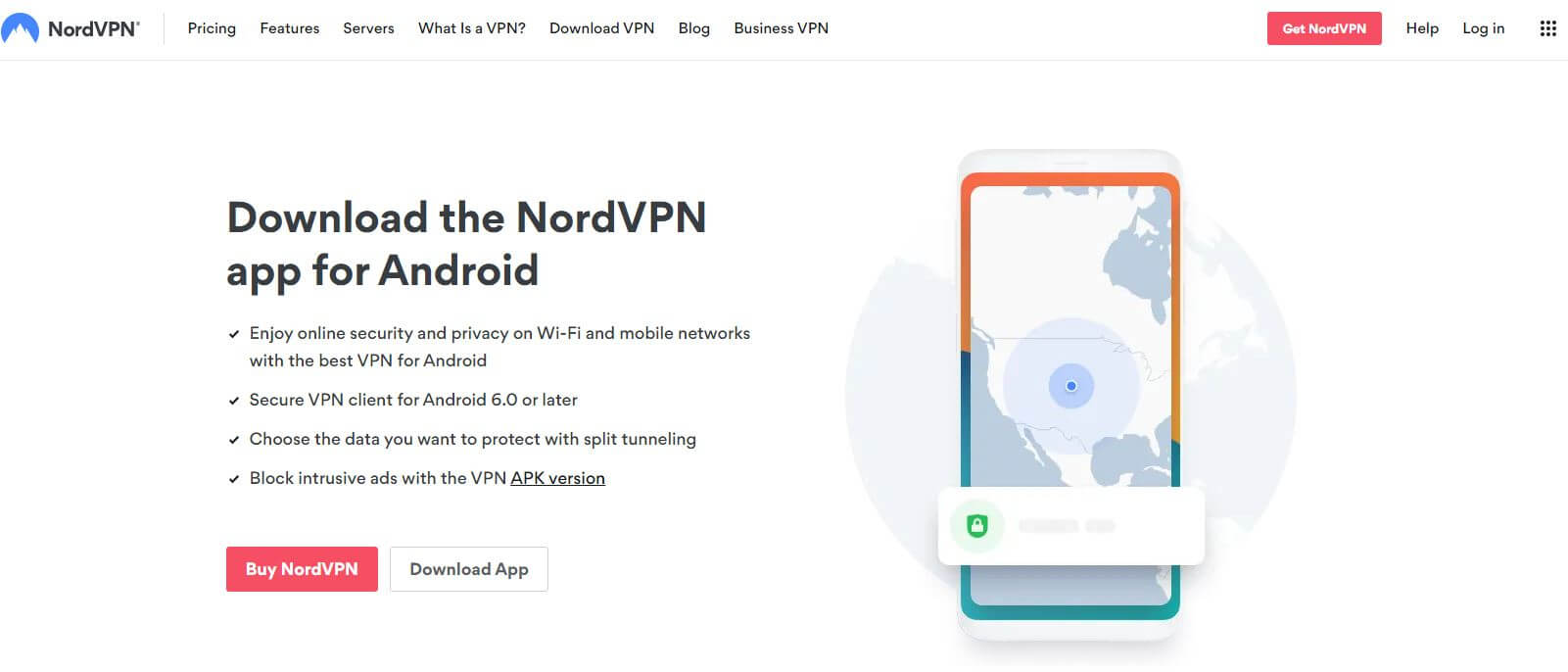**Caption:**

This webpage advertises the NordVPN app for Android, despite being viewed on a desktop platform. The NordVPN logo—a blue circle with a white mountain—is prominently displayed in the top left corner. Adjacent to the logo, the navigation bar includes options for Pricing, Features, Services, What is a VPN, Download the VPN, Blog, and Business VPN. To the far right, users can find links for Get NordVPN, Help, Login, and additional menu options.

The main content on the page highlights instructions for downloading the NordVPN app for Android, emphasizing the benefits of online security and privacy on Wi-Fi and mobile networks. The app supports Android 6.0 or later and offers features like split tunneling to choose specific data to protect and an ad-blocker in the VPN APK version. Users have the option to either buy NordVPN or simply download the app.

To the right of this information is an illustrative graphic: a world map centered on North America with a cell phone resting on it, symbolizing secure protection with NordVPN, represented by a lock icon.